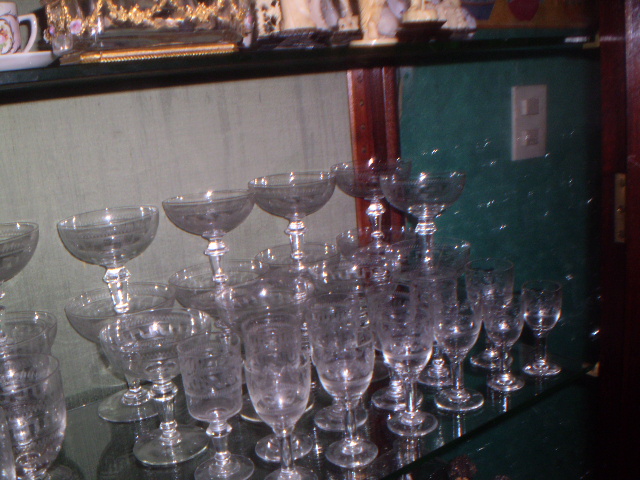The image showcases an elegant display of various stemmed glassware meticulously arranged on a shelf. In the foreground, there are rows of clear glasses, including wine glasses, cocktail glasses, and champagne glasses, with distinctive features such as fluted tops and bases. The glasses are stacked in two levels, particularly in the last row, where champagne-style glasses are nested within each other. The shelf is made of black wood, and above it, another shelf holds an assortment of knickknacks, including teacups, saucers, and porcelain figurines. The background incorporates a light green fabric-type wallpaper that transitions to a darker green with a wooden trim separating the two shades. The setting is further detailed with an electrical outlet on the darker green section of the wallpaper, adding to the intricate and sophisticated backdrop of the display.